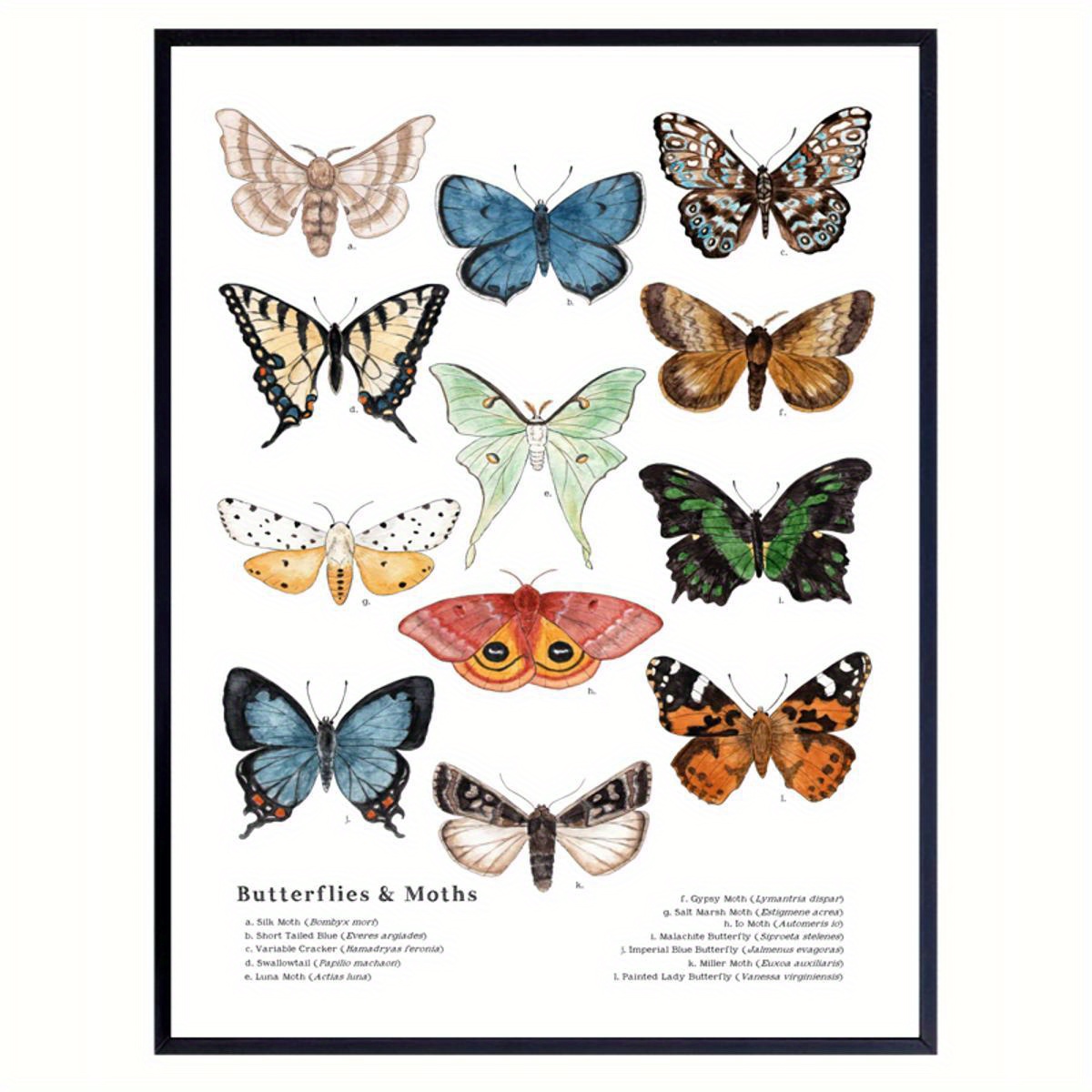The image depicts a beautifully illustrated page featuring a diverse array of butterflies and moths, framed by a quarter-inch black border. The page is white and split into three columns, each column showcasing a series of intricately hand-drawn, colorful specimens. 

- In the left column, the sequence begins with a brown striped moth at the top, followed by a tiger swallowtail butterfly, another moth beneath it, and ending with a blue swallowtail butterfly.
- The central column showcases a blue butterfly at the top, descending to a green luna moth, followed by a sphinx moth with pinkish wings and orange eye spots, and concludes with a nondescript brown moth at the bottom.
- The right-hand column starts with an ornately patterned butterfly displaying hues of brown, blue, and white. Below it is a brown moth, then a green swallowtail butterfly, and finally, an orange fritillary butterfly with orange spots.

Each butterfly and moth is numbered, and there is a key beneath the illustrations that describes their types, which includes species like the silk moth, luna moth, and gypsy moth, though the text is too tiny to read clearly. The detailed illustrations highlight a multitude of colors and intricate designs, showcasing the artist's skill and making the image resemble a well-crafted poster or framed artwork of butterflies and moths.